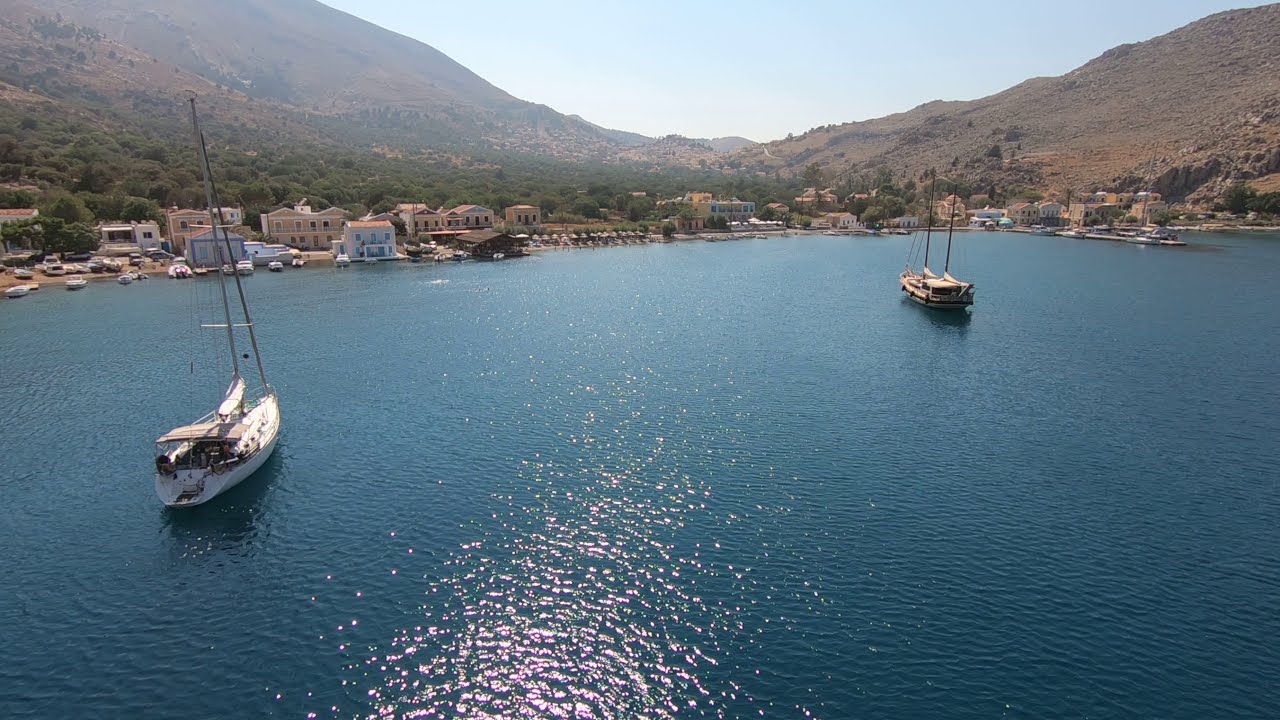This photograph captures a picturesque outdoor scene of a tranquil lake on a bright, sunlit day with clear, blue skies. The lake's deep blue waters shimmer under the sunlight, with gentle waves visible. In the center of the water, two sailboats float calmly; the one on the left, closer to the camera, is white, while the one on the right, further away, is brown. The expansive shoreline, spanning the entire top part of the image, features a variety of older structures and buildings. To the right side of the shoreline, there is a dock and several other boats moored. In the far distance, rolling hills create a scenic backdrop with a valley in the center, all blanketed by a light blue sky. The predominant colors in the image are brown, tan, green, blue, white, and hints of black and gray, delivering a serene and timeless lakeside landscape.